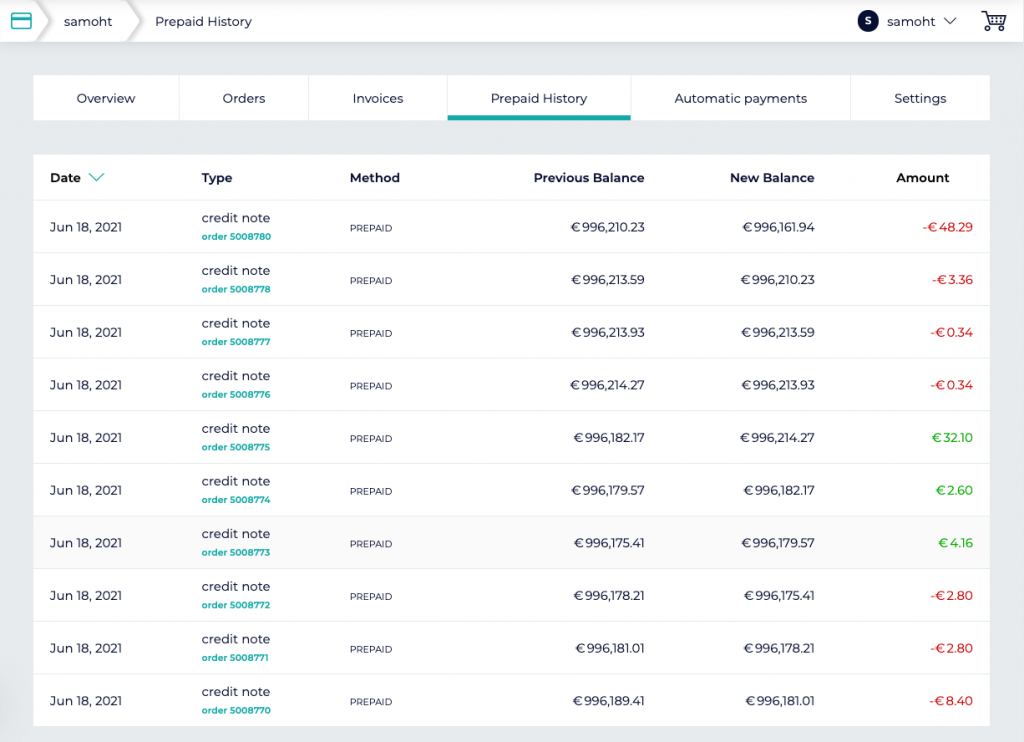This is an annotated screenshot detailing a series of credit note transactions for the user "Samholt" within a prepaid history application. At the top of the screenshot, "S-A-M-O-H-T" is displayed prominently. To its right, the title "Prepaid History" is shown. Below this, a circle containing the letter "S" represents the user icon, next to which "Samholt" is written. There is a dropdown arrow and a shopping cart icon beside the user's name.

The transactions listed are as follows:
- **June 18, 2021**: Credit Note, Method Prepaid
  - Previous Balance: $996,210.23
  - New Balance: $996,161.94
  - Amount: -$48.29
- **June 18, 2021**: Credit Note, Method Prepaid
  - Previous Balance: $996,213.59
  - New Balance: $996,210.23
  - Amount: -$3.36
- **June 18, 2021**: Credit Note, Method Prepaid
  - Previous Balance: $996,213.93
  - New Balance: $996,213.59
  - Amount: -$0.34
- **June 18, 2021**: Credit Note, Method Prepaid
  - Previous Balance: $996,214.27
  - New Balance: $996,213.93
  - Amount: -$0.34
- **June 18, 2021**: Credit Note, Method Prepaid
  - Previous Balance: $996,182.17
  - New Balance: $996,214.27
  - Amount: +$32.10

The transaction history continues beyond the listed entries, providing a clear, detailed view of account activities for "Samholt."